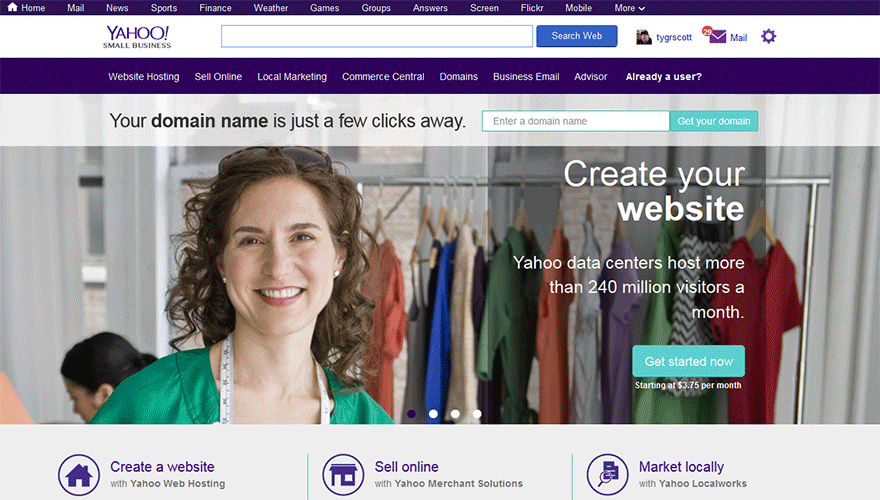This screenshot of Yahoo.com showcases a promotional banner encouraging users to create their own website. Central to the design is a prominent photograph featuring a smiling Caucasian woman with curly brown hair, dressed in a green top or dress, and a tape measure draped around her neck. The background suggests she is a seamstress, as it displays a rack of clothing. 

Above her is a toolbar featuring sections like Home, News, Sports, Finance, Weather, Games, Groups, Answers, Screen, Flickr, Mobile, and more, alongside icons for Mail, Profile, and Settings. 

Beneath the title "Create Your Website," it mentions, "Yahoo data centers host more than 240 million visitors a month. Get started now. Starting at $3.75 per month." There is also a search bar for checking the availability of domain names with a button labeled "Get Your Domain."

Below her picture, a purple option prompts users to "Create a Website with Yahoo Web Hosting." Another section encourages users to "Sell Online with Yahoo Merchant Solutions," and an adjacent purple icon offers the option to "Market Locally with Yahoo Localworks."

Overall, the page is a comprehensive guide to setting up a website, emphasizing ease of use and affordability, while picturing a user-friendly interface for domain and website management.